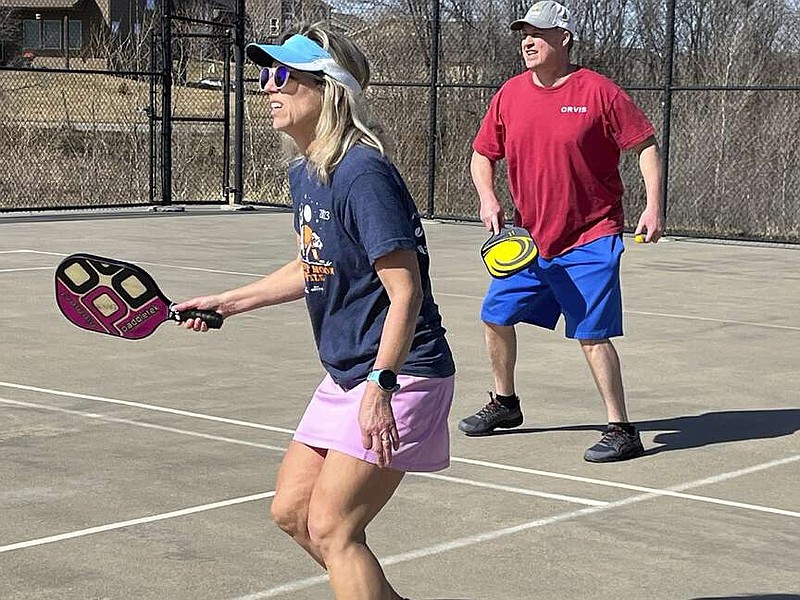In the photograph, a couple is engaged in a game of pickleball on a large court, reminiscent of a tennis court but equipped with smaller paddles instead of traditional rackets. The woman in the foreground is distinguished by her blonde hair, black t-shirt, pink tennis skirt, and a blue and white visor paired with sunglasses. She also has a smartwatch and wields a pink and black paddle. Behind her, the man is attired in a light-colored baseball cap, a red t-shirt with an indistinct graphic, blue shorts, and black sneakers, holding a yellow and black paddle. They are within a fenced-in area, and the background showcases a wintry, wooded environment with sparse trees and bushes, possibly suggesting a public park. They both appear to be anticipating the return of the ball, intently focused on the game.